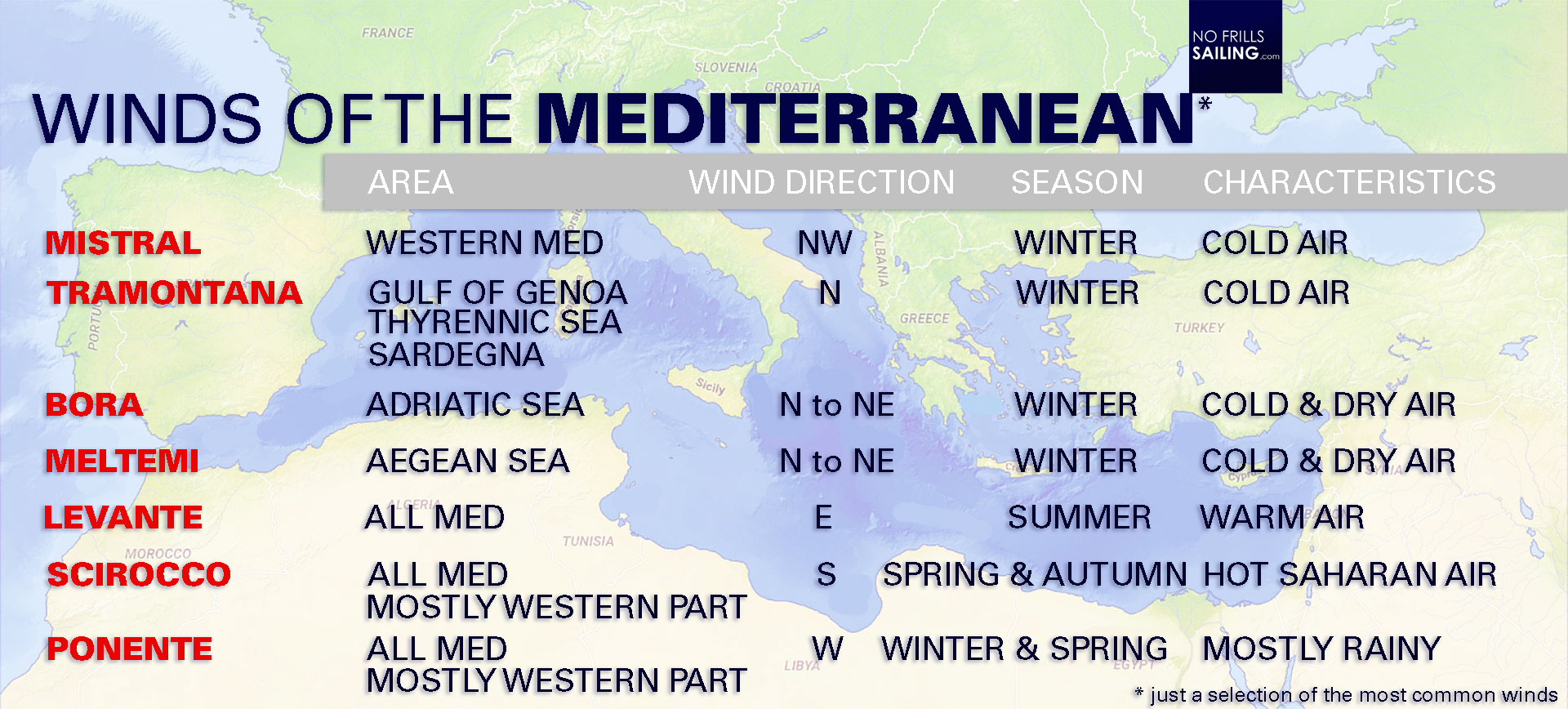The image is a horizontally aligned rectangular map depicting various countries around the Mediterranean Sea. Prominent features include a title in all caps black letters at the top left that reads "WINDS OF THE MEDITERRANEAN," with "Mediterranean" in bold. Just above the second 'N' in "Mediterranean," a small black square features the logo "NO FRILLS SAILING." The map itself displays green landmasses against bluish-gray water bodies.

On the left side of the image, red all-caps text lists the names of seven winds: "MISTRAL, TRAMONTANA, BORA, MELTEMI, LEVANTE, SIROCCO, and PONENTE." Below the title, a gray rectangular area contains a table with white headers, listing "AREA," "WIND DIRECTION," "SEASON," and "CHARACTERISTICS" from left to right. Each category is populated with black text detailing specific information about each wind:

- **Mistral:** Western Med, Northwest, Winter, Cold air.
- **Tramontana:** Gulf of Genoa, North, Winter, Cold air.
- **Bora:** Tyranic Sea, North to Northeast, Winter, Cold and dry air.
- **Meltemi:** Sardegna, North to Northeast, Winter, Cold and dry air.
- **Levante:** Adriatic Sea, East, Summer, Warm air.
- **Sirocco:** Aegean Sea, South, Spring and Autumn, Hot Saharan air.
- **Ponente:** All Med, West, Winter and Spring, Mostly rainy.

At the bottom of the image, an asterisk notes that this is just a selection of the most common winds.